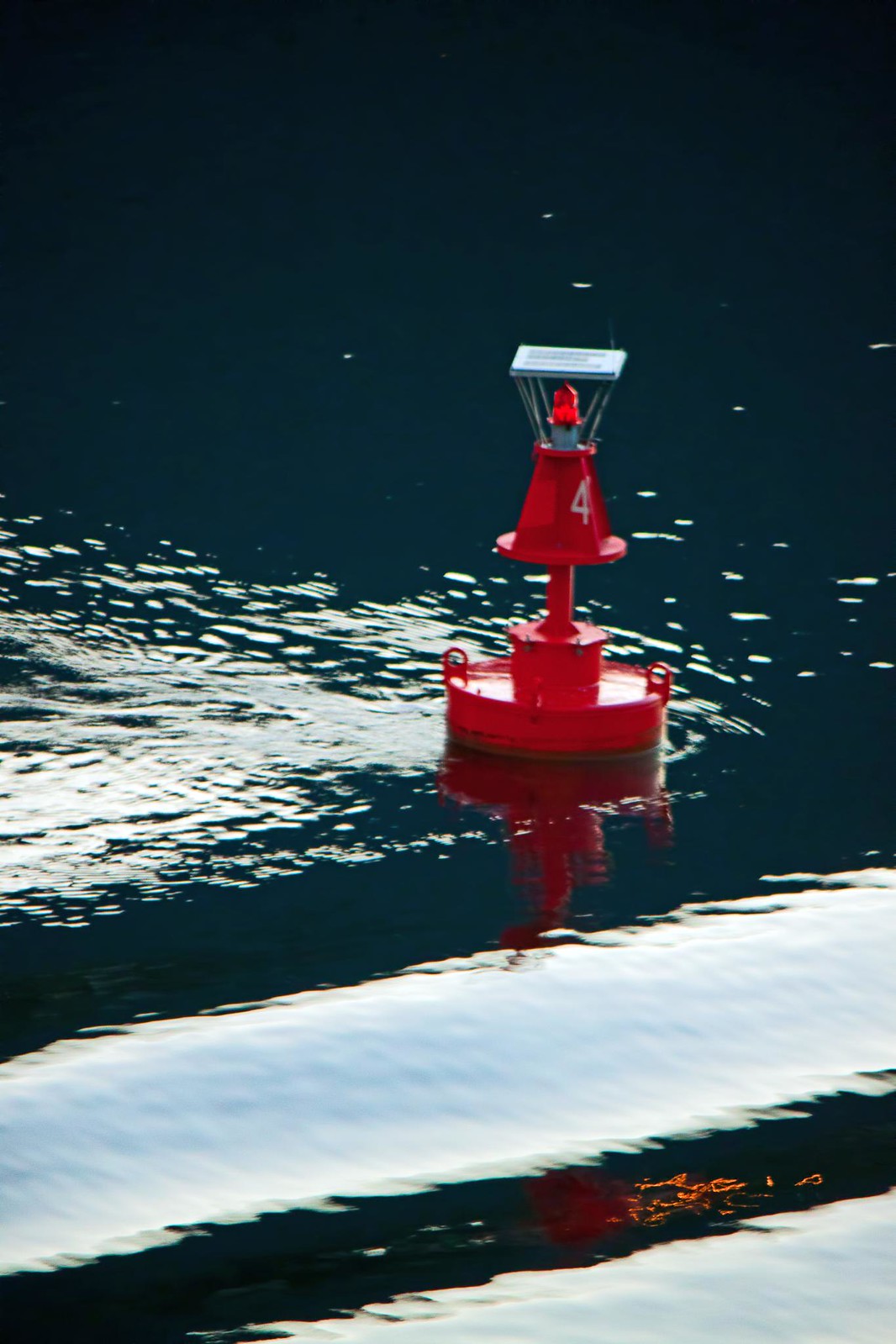In this color photograph, taken in portrait orientation, a red navigational buoy is prominently featured floating serenely on calm, dark water. The tranquil surface of the water creates stunning reflections, including a triangle of sunlight pointing towards the buoy and broad swaths of sunlight reflecting diagonally across the bottom of the image. The buoy, designed for maritime navigation, showcases a complex structure. It consists of a larger round base, a cylindrical middle section, and a narrower pole. Atop the pole sits a red, cone-shaped figure reminiscent of a traffic cone, marked with a white number "4." Above this, there is a safety light, likely powered by a solar panel, housed under a flat top for protection from rain. The entirety of the buoy, including the light and its protective cover, is in red, with the number "4" standing out in stark contrast. This buoy likely serves both illumination and signaling purposes, aiding boaters in navigating safely through the channel.